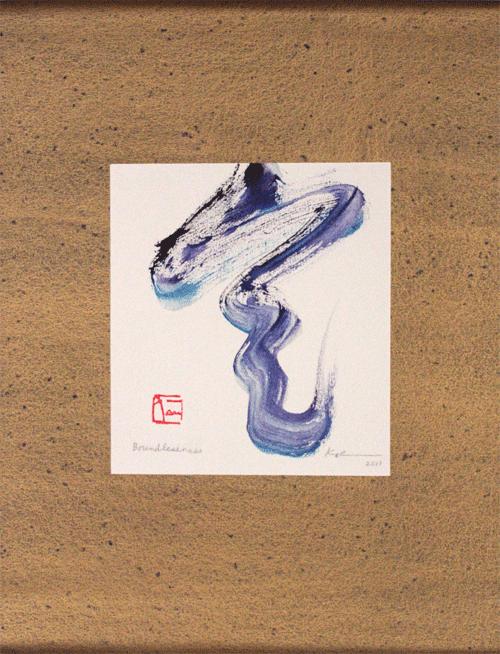In the center of the image, there's a piece of white paper adorned with an abstract painting, placed on a textured brown surface that resembles either wood or a gravelly rubberized material. The painting is characterized by sweeping brush strokes that form a spiral pattern, featuring a diverse palette of colors including light brown, black, white, red, gray, purple, and various shades of blue and teal. The artwork, which appears to be hand-painted, gives the impression of a snake whose head was never completed, with its body painted in black, purple, light purple, and blue. At the bottom left corner of the paper, there is a small red logo and some text, while at the bottom right corner, additional writing and some numbers are visible. However, none of the text is legible. This abstract piece could be an amateur painting, possibly hung on a wall in a home setting.